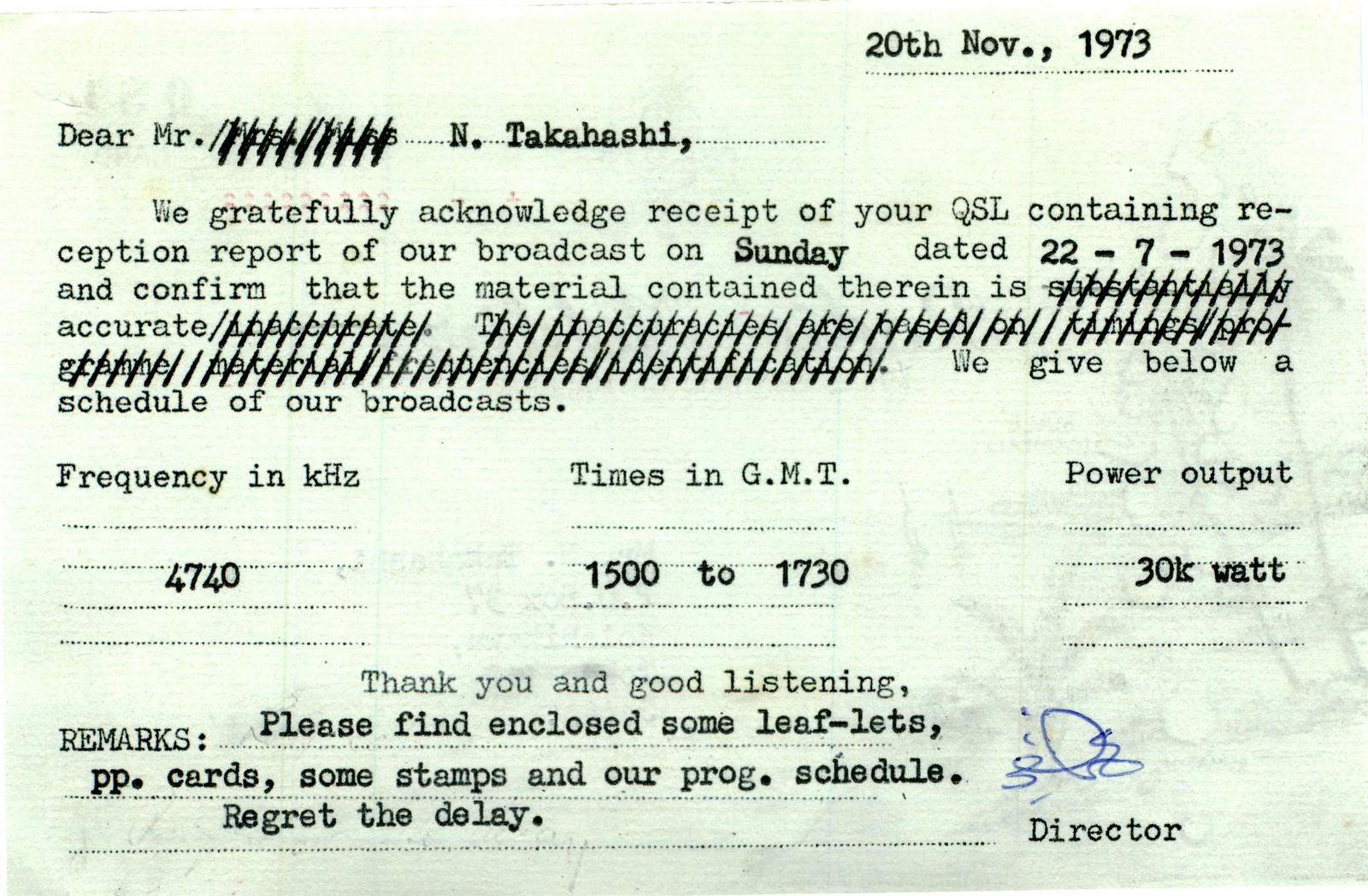The image depicts a QSL report for radio frequency acknowledgement, printed on a greenish-white postcard-sized piece of paper. Dated 20th November, 1973, it is addressed to Mr. N. Takahashi. The text acknowledges the receipt of Mr. Takahashi's QSL-containing reception report for a broadcast on 22nd July, 1973, confirming the accuracy of the report despite certain sections being marked out with slashes. It provides a broadcast schedule with frequencies at 4740 kHz, airing from 1500 to 1730 GMT, with a power output of 30kW. The note also mentions enclosed items such as leaflets, PP cards, stamps, and a program schedule, and extends apologies for the delay. The letter ends with a courteous message from the Director, accompanied by the Director's signature.